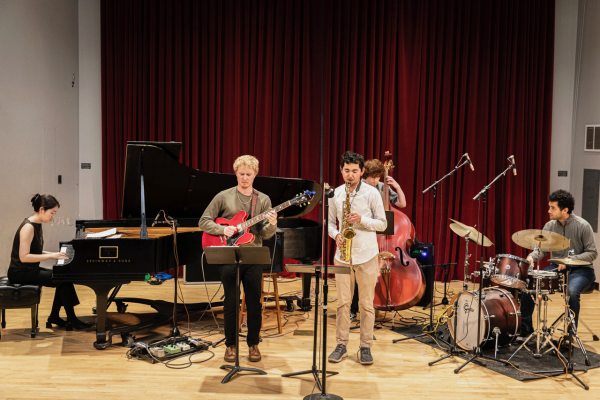The photograph captures a detailed scene of a band rehearsal in a music hall, possibly at a school or theater. Center stage is a male guitarist with light blonde hair, wearing a tan shirt, black pants, and brown shoes. He is playing a red electric guitar and intently studying sheet music on a stand in front of him. Adjacent to him is a saxophonist, dressed in a white button-down shirt and brown pants, with dark hair, engrossed in his music notation as he plays his saxophone. 

To the right of the saxophonist and guitarist, a young man, wearing jeans and a gray long-sleeve sweater, is seated at a drum set. The brown drum kit is adorned with hanging microphones, indicating a professional setup, as he looks towards his bandmates, likely to synchronize his rhythm.

Slightly behind the saxophonist, another young man is playing an upright bass, partially obscured but visibly plucking the strings of the large instrument with his fingers.

On the far left, an Asian woman dressed entirely in black, sits at a grand piano. The black, open-top piano contrasts with the wooden floor and stands out against the backdrop. She is focused on her playing, adding to the harmonic ensemble.

The stage is set with audio equipment and cables scattered around, showcasing the technical setup. The background features long burgundy curtains against white walls, contributing to the formal and focused atmosphere of the band practice.